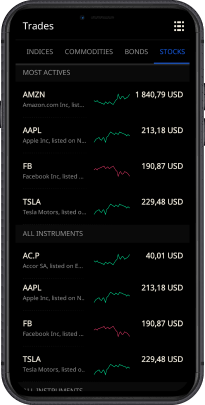A screenshot featuring a black background presents an assortment of financial data. This data includes trades, invoices, commodities, bonds, and stocks, primarily displayed in a vivid blue interface. The section titled "Most Actives" lists several major companies with their stock tickers and corresponding performance indicators. 

- **Amazon (AMZN)** is represented by a green upward line, with its stock price noted at **1,840.79 USD**.
- **Apple (AAPL)** also shows a green upward trend, with a stock price of **213.18 USD**.
- **Facebook (FB)** is depicted with a red downward line, indicating a stock price of **190.87 USD**.
- **Tesla (TSLA)** has a green upward line, with a stock price of **229.48 USD**.
- Another entry, **AC.P**, shows a green upward line with a value of **4,001 USD**.

Each stock's performance is visually indicated by green lines for gains and red lines for losses. The caption concludes with a message of appreciation: "Thanks for watching!"